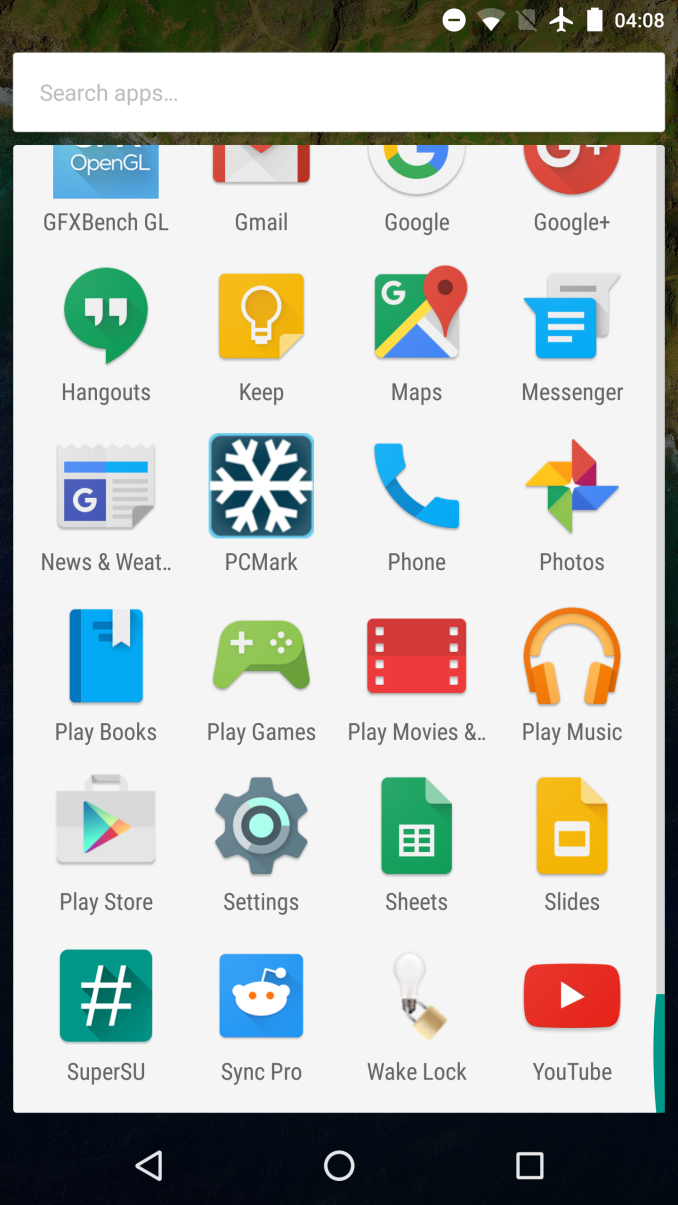Screenshot Description:

The screenshot, set against a white background, displays a device's home screen with the current battery level at 40%. At the top, the status bar shows an airplane mode icon. Below this, there's a prominent search bar labeled "Search apps..." indicating functionality to search the device's applications.

The home screen features a variety of application icons arranged in rows. The visible apps include:

1. GFXBench GL
2. Gmail
3. Google
4. Google Plus
5. Hangouts
6. Keep
7. Maps
8. Messenger
9. News
10. Weather (abbreviated as "W E A T...")

Additional apps listed are:
11. PC Mark
12. Phone
13. Photos
14. Play Books
15. Play Games
16. Play Movies
17. Play Music
18. Play Store
19. Settings
20. Sheets
21. Slides
22. SuperSU (abbreviated as "S U")
23. Sync Pro
24. Wake Lock
25. YouTube

At the bottom of the screen is a black navigation bar, displaying three white icons: a left arrow (back button), a circle (home button), and a square (recent apps button).